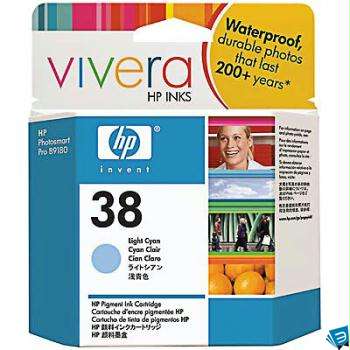The image showcases a detailed package for an HP ink cartridge. At the top of the package, is a small hole designed for hanging on store hooks. Prominently displayed in colorful letters at the top is the word "Vivera," followed by "HP Inks." Adjacent to this text is an orange section that emphasizes the ink's qualities: "waterproof, durable, photos that last 200 plus years." Below this, the predominantly white and light blue packaging features the HP Invent logo on the left side. Just below the logo, the cartridge number "38" and the color "Light Cyan" are clearly indicated. To the right, a series of vibrant photos demonstrate the ink's quality, depicting a smiling woman, a clear sky, pedestrians, and oranges. The right side panel of the box is also visible and includes some additional text in black on a white background.